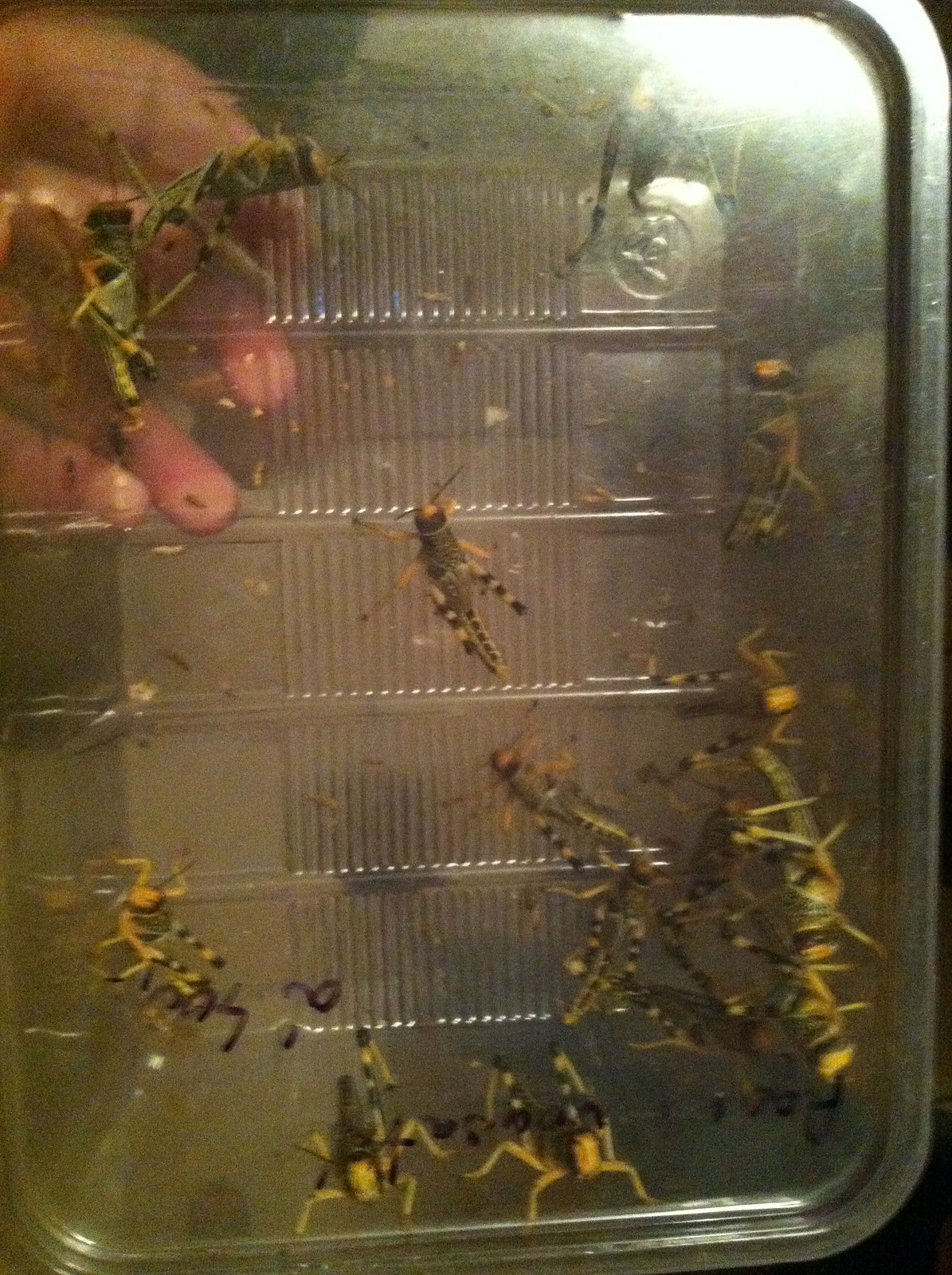The indoor color photograph features a clear, rectangular plastic tray held upright by a hand visible in the upper left corner. The tray, somewhat resembling a take-out container, contains numerous fully-grown grasshoppers predominantly in green with tan legs and striping on their bodies. These grasshoppers are dispersed across the tray, with the majority clustered in the lower right portion and a few distributed in the upper left near the supporting hand. One solitary grasshopper occupies the center. The image is dimly lit and slightly out of focus, making details indistinct. Faint black marker lettering appears on the tray, though only partially legible, showing fragments such as "A" and "S." The camera angle suggests a view from below, as if the camera were positioned on the floor, emphasizing the transparency of the tray and the insects' legs.